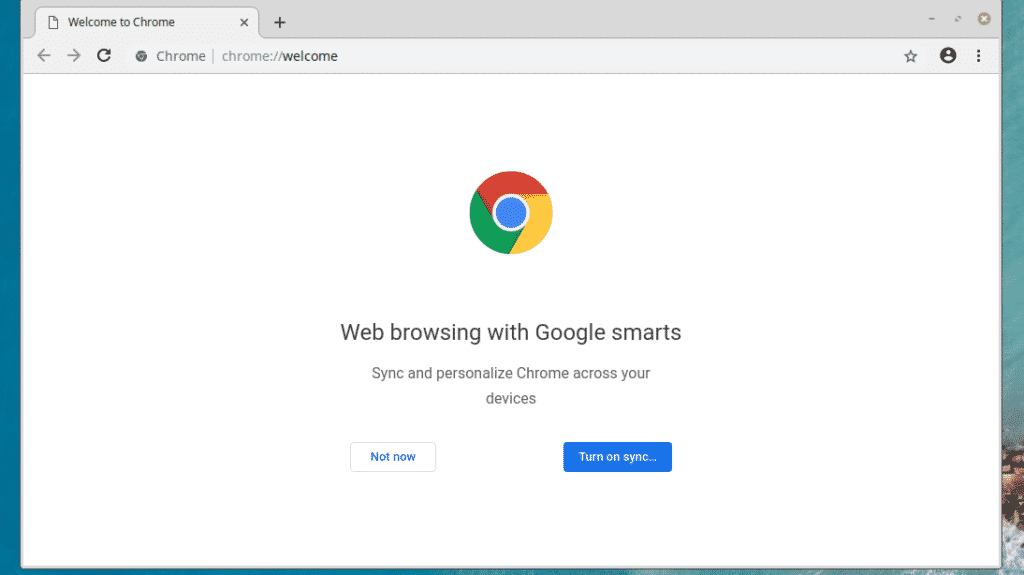Screenshot of a partially open Google Chrome welcome page window. The window is not maximized, revealing portions of a blue home screen along the top, left, and right edges. The welcome page is white, prominently displaying the Google Chrome logo: a blue circle encircled by a donut-shaped ring segmented into red, yellow, and green sections. Below the logo, the text reads: "Web browsing with Google smarts. Sync and personalize Chrome across your devices." 

At the bottom, there are two buttons. The grey "Not now" button is on the left, and the highlighted blue "Turn on sync" button is on the right. The URL bar at the top shows "chrome://welcome" and on the right-hand side of the URL bar, there are icons for a star (to bookmark), the user's profile, and a vertical three-dot menu.